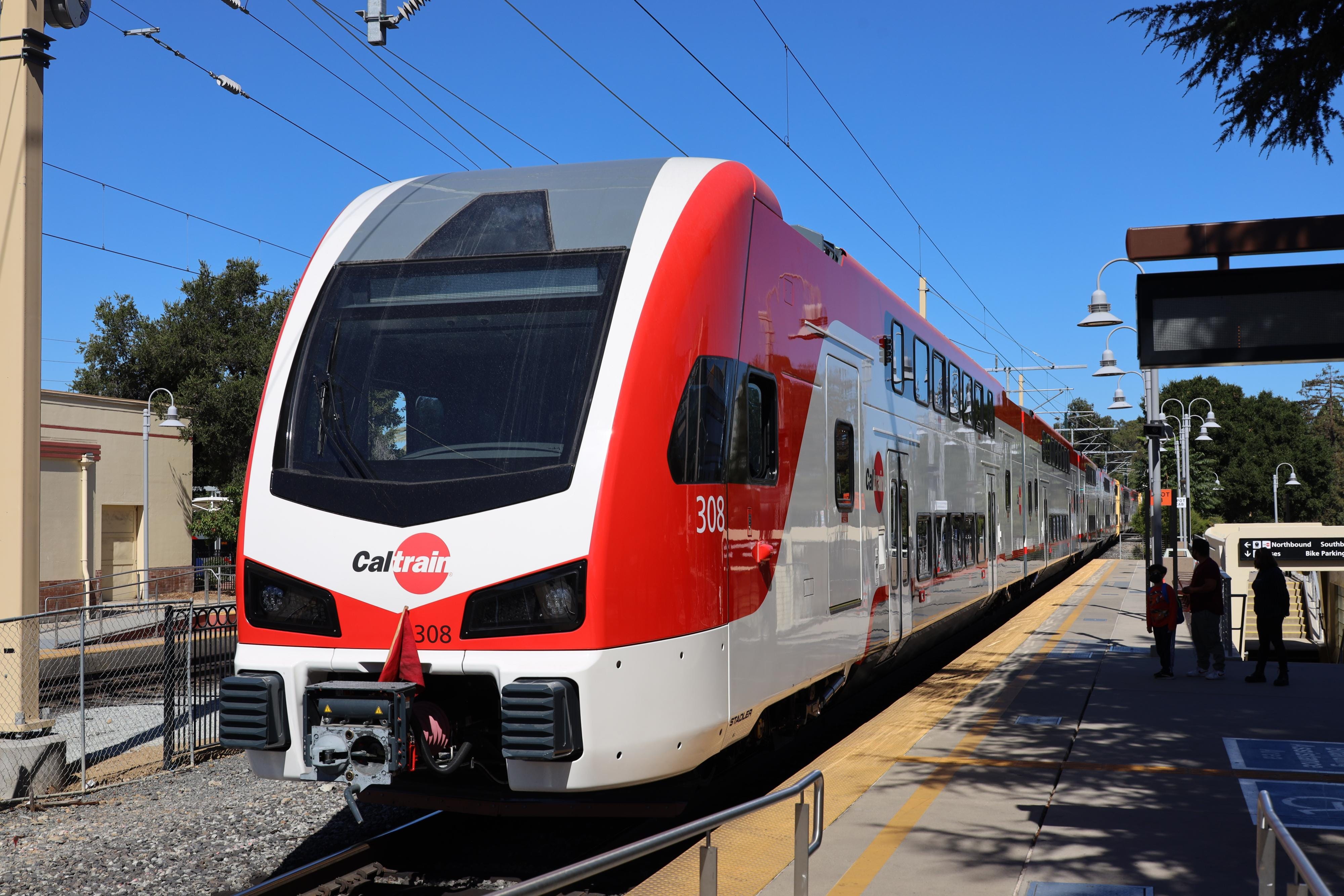The photograph captures a sleek, modern train with the logo "Cal Train" prominently displayed on its front, indicating it might be from California. The train, numbered 308, features a red and white color scheme, with the red accent running along the top and front of the vehicle. It sits stationary on a platform made of cement, adorned with distinct brownish gold caution stripes, and bordered by gray gravel alongside the tracks. The platform is well-lit by evenly spaced lamplights, and a staircase is visible to the right. Overhead, an intricate network of wires suggests that the train is electrically powered, with connections extending upwards to these wires. In the foreground, three silhouetted figures—two adults and a child—stand in the shadows, seemingly waiting to board. The bright blue sky serves as a backdrop, contrasting with the darkened glass of the train's sleek, streamlined exterior. In the distance to the left, there's another building with a lamp in front of it, framed by some trees behind.